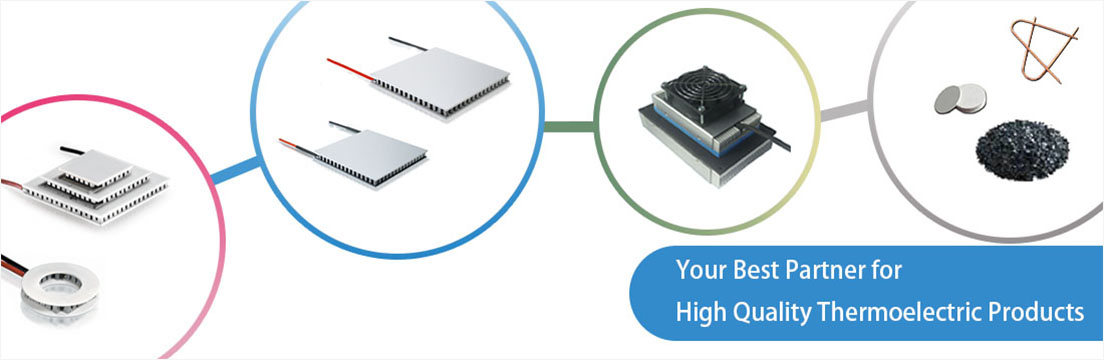The image appears to be a detailed diagram from a guidebook or textbook showcasing various electronic products. It features four interconnected circles, each with distinct colored borders: fuchsia pink, blue, green, and gray. Each circle contains a photo of different electronic components. The fuchsia pink circle on the far left houses what seem to be computer chips. This connects to the blue circle, which also contains computer chip-like objects, via a small blue line. A green line links the blue circle to a green-bordered circle, which includes another chip. Finally, a gray line stretches to a partially visible gray-bordered circle containing a pile of crushed rock or ash, thin batteries, and what appear to be two open paper clips laid perpendicularly. Additionally, the image includes two flat gray boxes with ventilation holes, possibly for air circulation, and either antennas or cords. One of these boxes resembles a tower with a ring-shaped device next to it. The bottom right corner of the image has a text tagline in white on a blue backdrop that reads, "Your best partner for high-quality thermoelectric products."